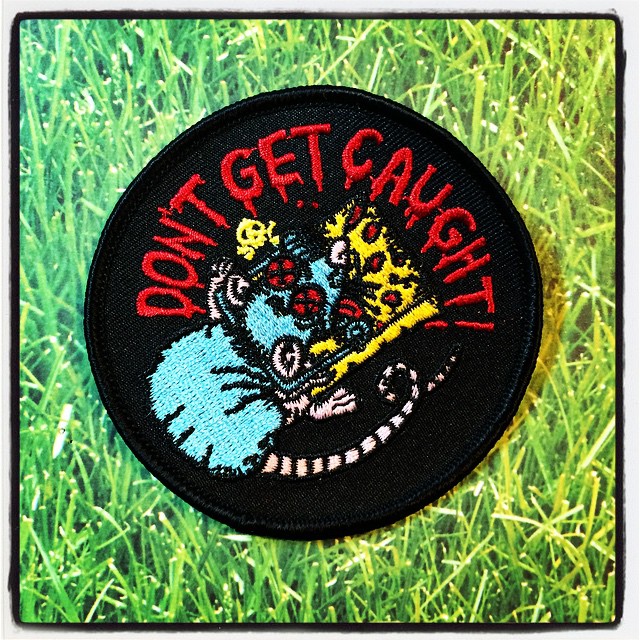This detailed photograph features a square-shaped image with a dark black border framing vibrant green grass illuminated by sunlight. Superimposed on the grass is an intricate, circular black patch reminiscent of those used by Girl Scouts, designed to be sewn onto fabric. The patch itself has "Don't Get Caught" embroidered in red across the top in a dramatic, bloody dripping font. At the center of the patch is an illustration of a blue rat with red eyes, a tan-colored tail with black and white stripes, and tan feet. The unfortunate rat is depicted caught in a yellow mousetrap, with the trap snapped shut around its neck. Adding to the macabre scene, the rat has its tongue hanging out, red X's marked over its eyes, and hints of blood, alongside small skull and crossbones symbols that suggest it met its demise. The green grass background adds a stark contrast to the dark theme of the patch, making the detailed elements of the embroidered badge stand out clearly.